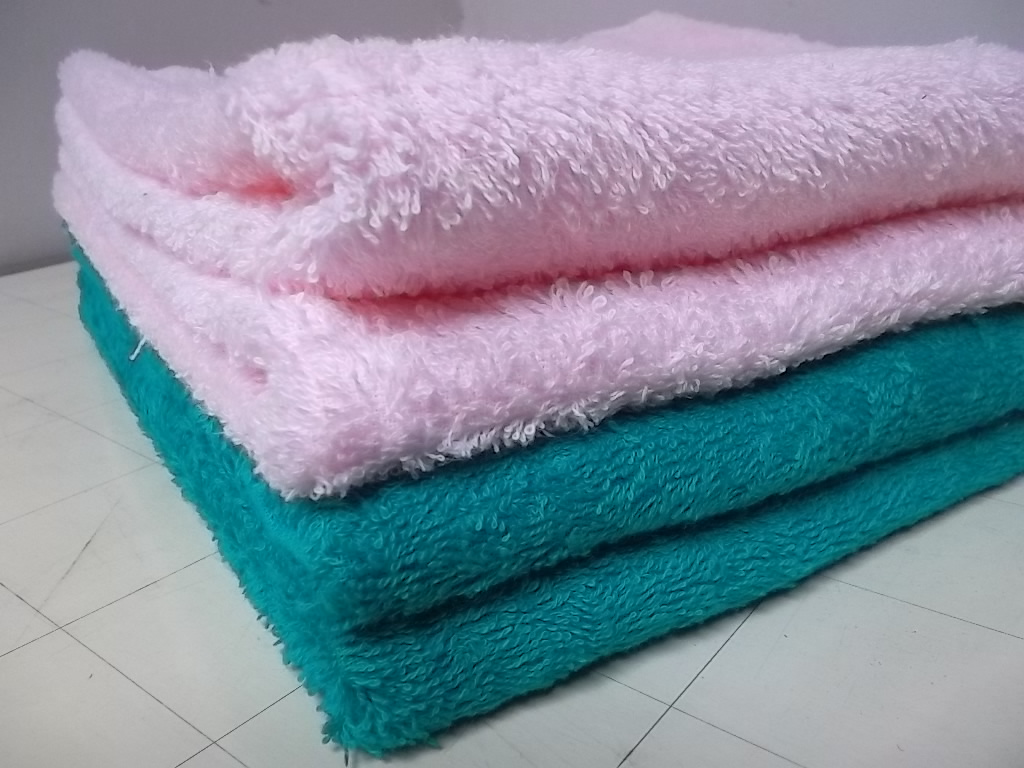This close-up photograph features a neatly stacked pile of four fluffy towels, arranged on a white, square-tiled countertop. The array shows a bird's-eye view of the towels, each folded in half lengthwise with the fold facing forward. The two towels at the bottom are a vibrant turquoise or teal color, while the two on top are a light pink hue. The towels have a visibly textured appearance with individual raised fibers, and the top pink towels appear slightly fuzzier than those beneath, possibly indicating a different brand or texture. The scene is set against a plain white wall, with the lighting casting a cool, white hue. The careful arrangement of the towels and their plush, inviting texture create a harmonious and soothing visual.